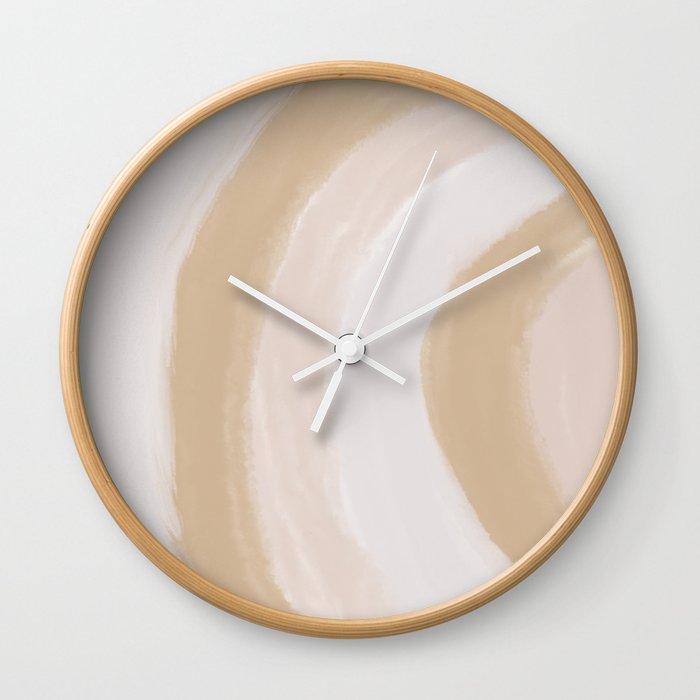This square image showcases a creatively designed analog wall clock, which stands out due to its elegant, light wood frame that might be polished birch or bamboo. The frame's subtle sheen highlights its nicely treated surface. The clock's face is uniquely adorned with a gradient of colors resembling a sideways rainbow, where curved stripes flow from left to right in a sequence of white, dark tan, light tan, white, dark tan, and light tan. The stripes create a visually appealing wave-like pattern across the clock's face. All three hands—the hour, minute, and second hands—are stark white, and the clock lacks any numerical markings, enhancing its minimalist aesthetic. The clock appears to display a time close to 9:05 and 15 seconds. In the background, the wall is a very light gray, subtly complementing the clock’s light and airy color scheme.